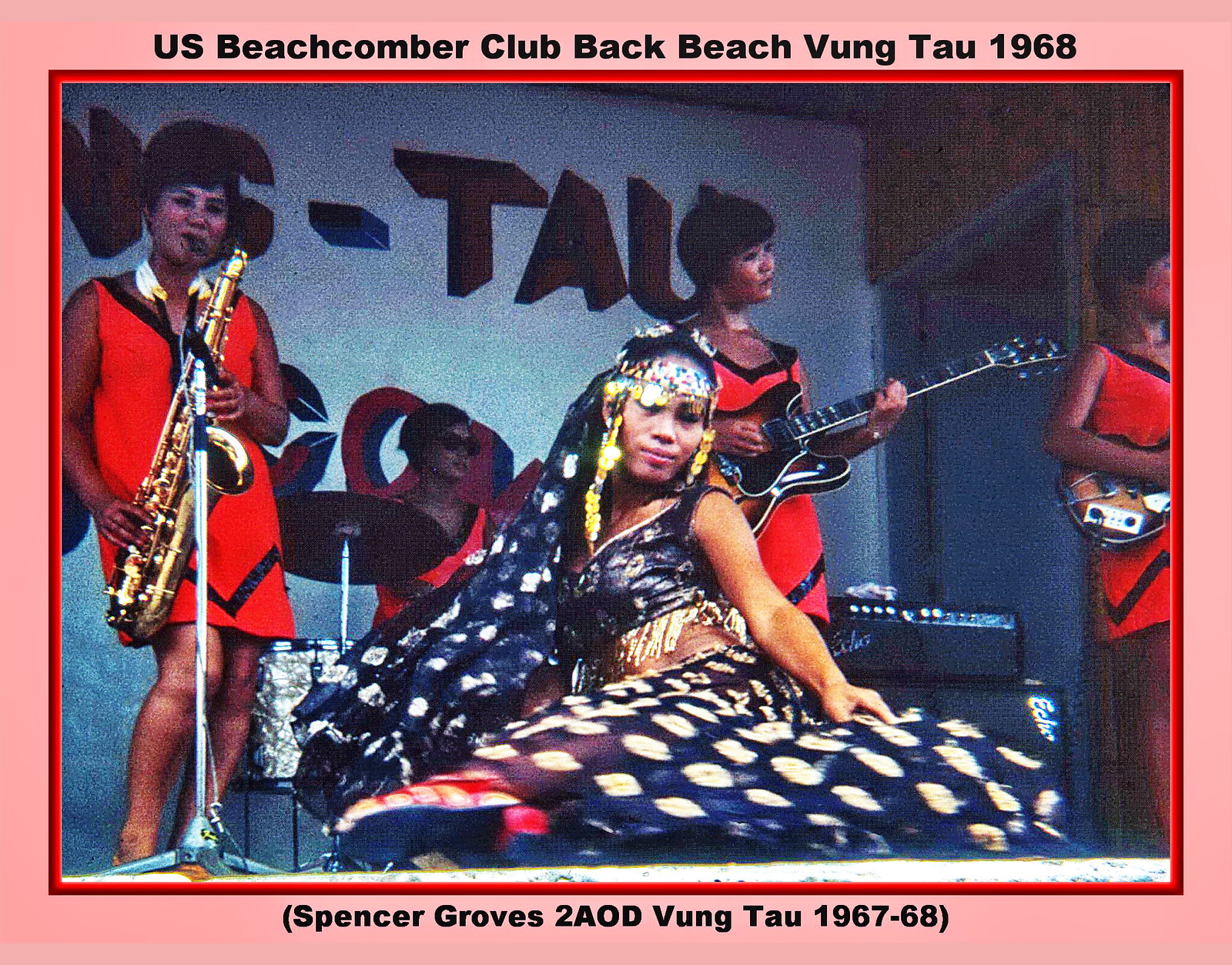The large, square image features a prominent pink border that frames a photograph with a red border. At the top, black text reads "U.S. Beachcomber Club, Back Beach, Vung Tau, 1968," and underneath, the caption "Spencer Groves, 2AOD, Vung Tau, 1967-68" is seen below the picture. The photo captures an all-female Vietnamese band performing on stage against a blue background adorned with black writing that partially spells "Vung Tau" in the upper left corner. In the foreground, a woman, dressed in an elaborate white and black dress with gold fringe and a matching long veil, sits on the stage floor. To her left, another woman in a red sleeveless dress with black trim plays the saxophone, while in the background, a drummer wearing sunglasses keeps the beat. On the right side of the stage, two women, also in red dresses and sporting short black hair, play guitars. The scene is vibrant and energetic, reflecting a 1968 musical event at the U.S. Beachcomber Club, likely providing entertainment for the troops stationed there.